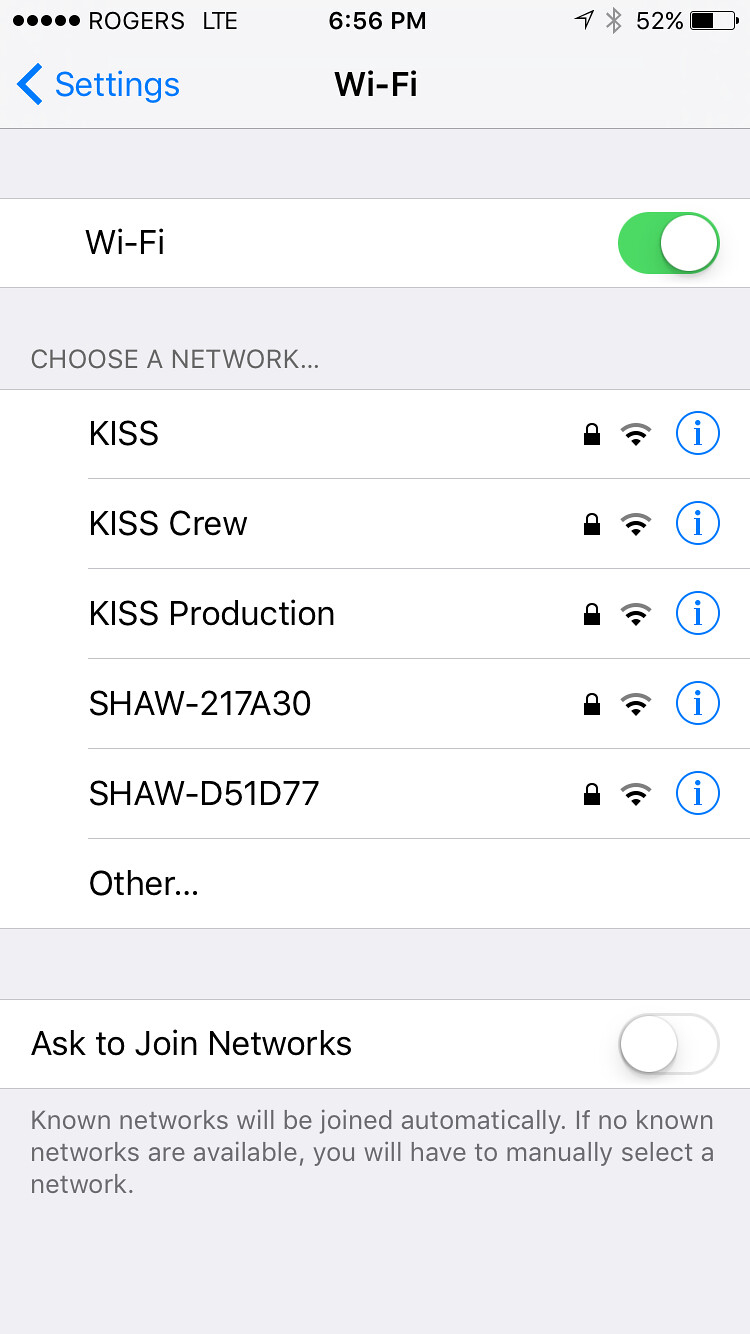The image is a screenshot taken from a phone displaying the Wi-Fi settings page. At the top, in black letters, it shows the time as 6:56 p.m. The battery level is at 52%, and the carrier is Rogers LTE, with these details aligned horizontally. Below this, there's a blue arrow on the left labeled "Settings" and a title that reads "Wi-Fi" with a green toggle switch indicating that Wi-Fi is turned on. Underneath, a section titled "Choose a Network" lists various Wi-Fi networks: KISS, KISS Crew, KISS Production, SHA-217A30, SHA-D51D77, followed by an "Other" option. Small lock icons appear next to the listed networks. Towards the bottom of the screen, there's an "Ask to Join Networks" section with its toggle switch turned off. Below this, in smaller gray text, it states, "No networks will be joined automatically. If no known networks are available, you will have to manually select a network."